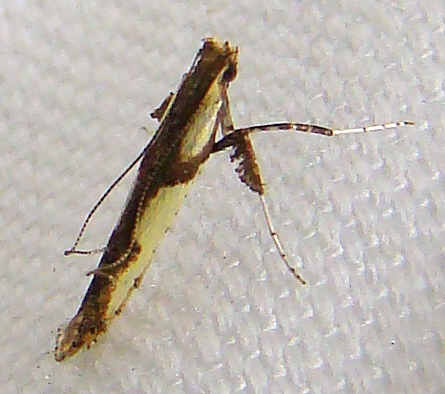This is a very detailed, close-up color photograph of a bug perched on a textured, off-white background that appears to be a man-made material, possibly fabric with a stitch pattern. The image is square in format and intentionally focuses on the intricate details of the bug. 

The bug itself seems to be a type of grasshopper or its larval stage, characterized by its very long, thin legs that appear sharp and pointy. It possesses four visible legs and extremely long antennas that extend to its rear. The body of the bug shows a distinct contrast in coloration, being very dark on the top and white on the bottom, with an orange-yellowish hue. The creature also has two visible eyes and hints of transparent wings that have not been spread.

You can almost see through parts of its legs into what looks like its skeletal structure. The detailed texture of the background contrasts with the delicate, almost alien features of the bug, adding a striking depth to this simple yet captivating nature photograph.